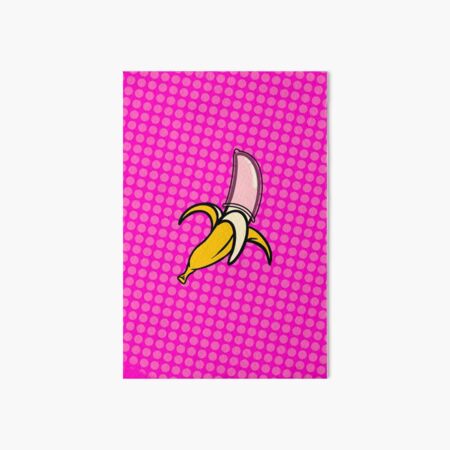In the center of a textured hot pink rectangle set against an off-white square background, a cartoon banana is prominently featured. The vibrant pink background is patterned with angled tiles of lighter pink circles and darker pink spaces in between, creating a striking visual effect. The banana itself is half peeled, revealing three distinct yellow peels parting at the bottom, exposing the soft flesh of the fruit above. The stem of the banana is positioned at the lower left corner, while the fruit points diagonally towards the upper right corner. The banana flesh, slightly tinted pink from the background, shows subtle details including three horizontal black lines, and the inside of the foremost peel is white, adding contrast and depth to the whimsical image.